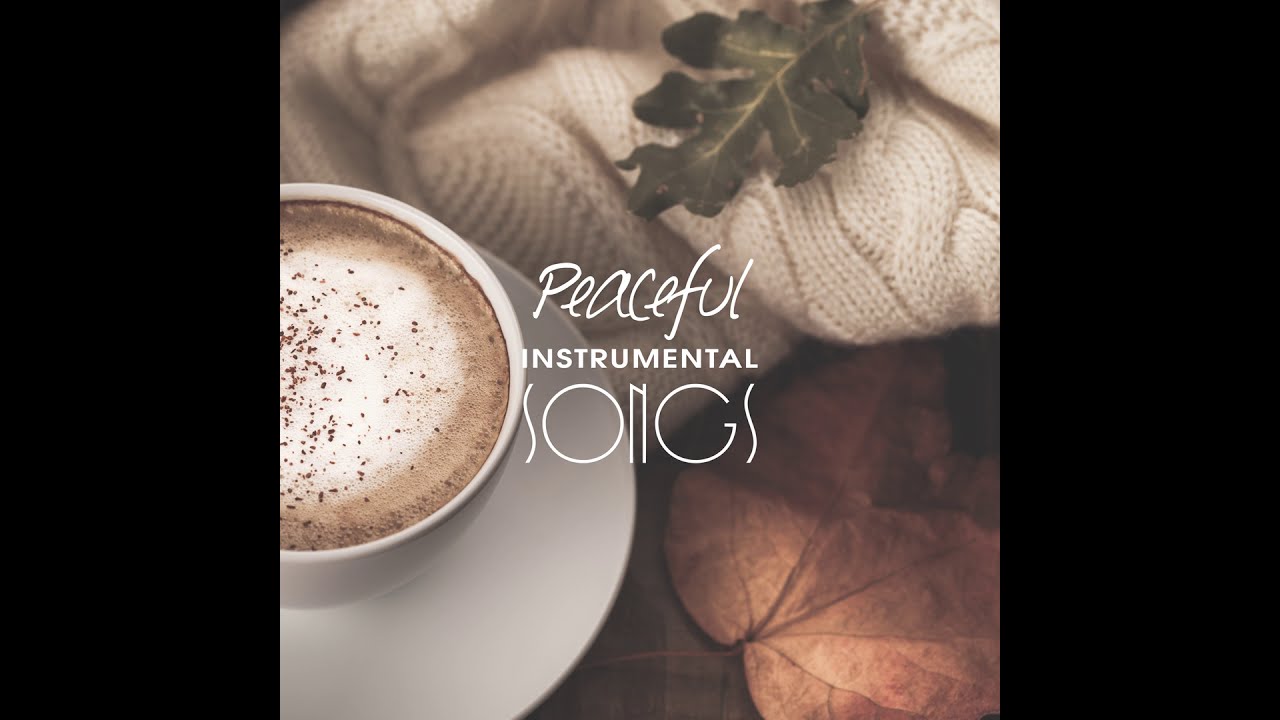The image is a cozy, warm-toned color photograph, likely designed as album art or playlist cover. Dominating the left-hand side is a cup and saucer, partially cut off, with a warm brown beverage that appears to be a latte or hot chocolate, topped with white foam and possibly a dusting of cinnamon or chocolate shavings. Adjacent to the cup on the right, there's a folded beige cable-knit blanket or sweater, adding to the inviting atmosphere. On top of this knitted fabric lies a green oak leaf, with a larger, broad brown leaf positioned below it. The center of the image features three lines of white text in varying fonts: the top line is in a flowing script, the middle line is in thin block capitals, and the bottom line is a modern, artsy style, all together reading "peaceful instrumental songs." The overall composition exudes a sense of autumnal warmth and tranquility.